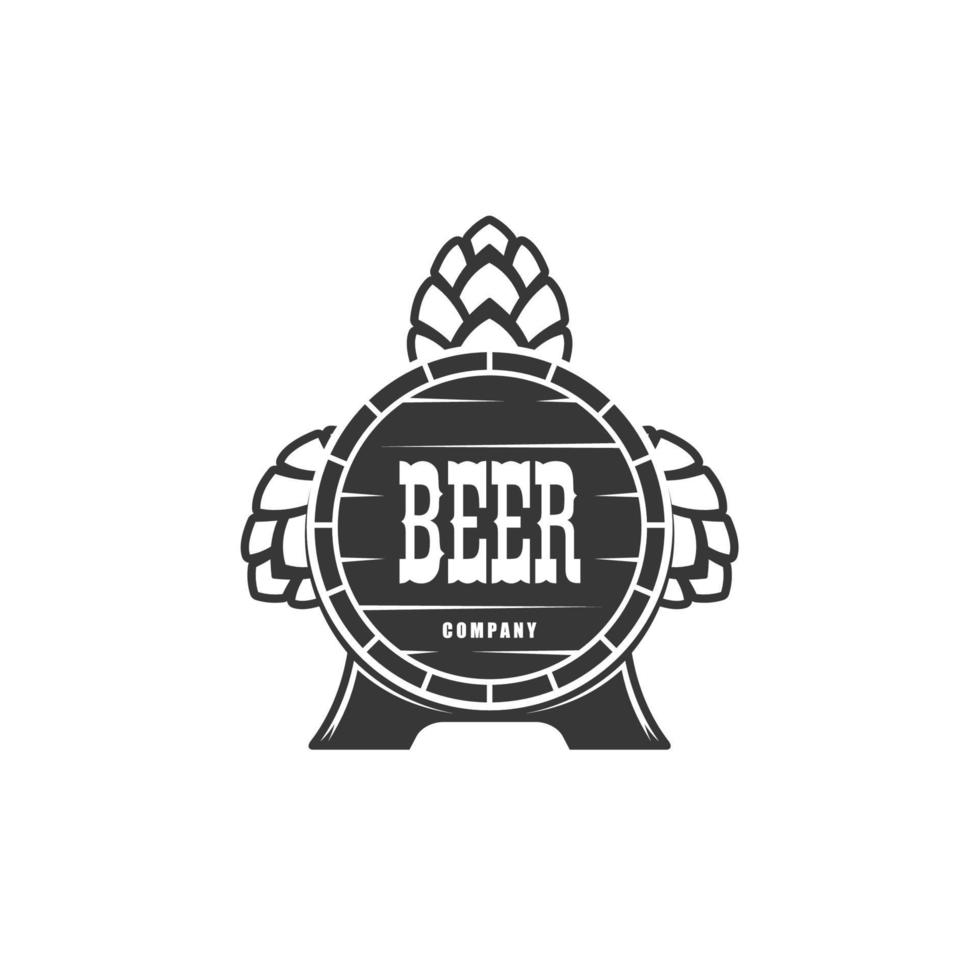The image depicts a circular logo rendered in black and white, likely that of a local beer company. Dominating the center of the logo is a stylized representation of a beer barrel, which seems to artistically double as the body of a turtle. The main feature of the barrel is the word "BEER" inscribed in large, bold, western-style uppercase letters, with the word "COMPANY" appearing in smaller, centered, white uppercase letters beneath it. Surrounding the turtle-shaped barrel are three graphic design elements that resemble pine cones, positioned at the top and on both sides, suggesting the turtle's head and arms. The bottom of the logo features a design akin to the base of the Eiffel Tower, acting as the turtle's legs or a stand for the barrel. The overall design, outlined in black on a white background, appears somewhat like a medallion or sign, effectively capturing the essence of the brand.